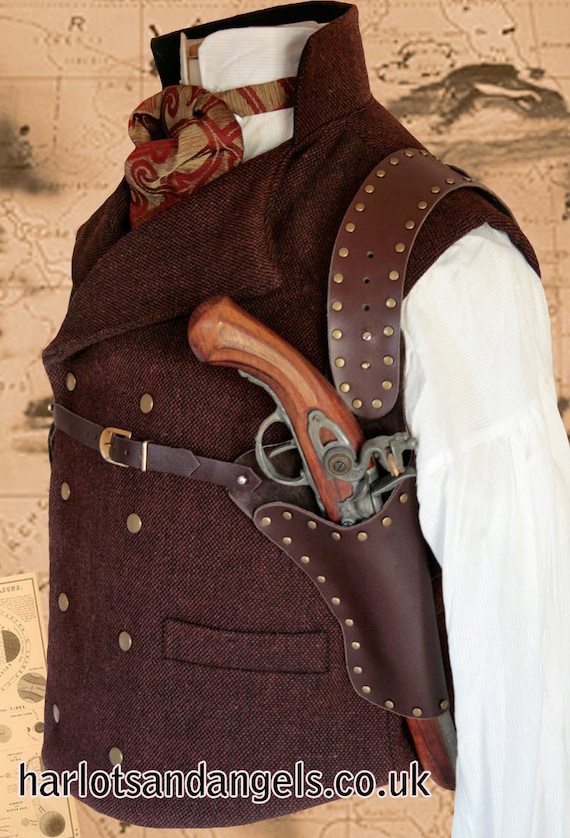The image displays a detailed Western-style costume set against a brownish map background adorned with black mountain ranges and outlines. The outfit features a long-sleeved white button-up shirt, partially visible with one sleeve fully displayed. Over the shirt is a dark reddish-brown tweed vest with brass buttons, four on each side, and an upturned collar that transitions into a popped-up back resembling a turtleneck. The neck is adorned with a beige and red scarf tied neatly. A leather strap is slung over the right shoulder, leading to a gun holster that holds a flintlock pistol, showcasing its wooden handle and steel trigger. Notably, at the bottom of the image, the text "harlotsandangels.co.uk" is printed in black lowercase with a white border, indicating the costume's brand. The intricate background, reminiscent of an old map with its sandy tint and dark embellishments, adds an authentic historical touch to the ensemble.